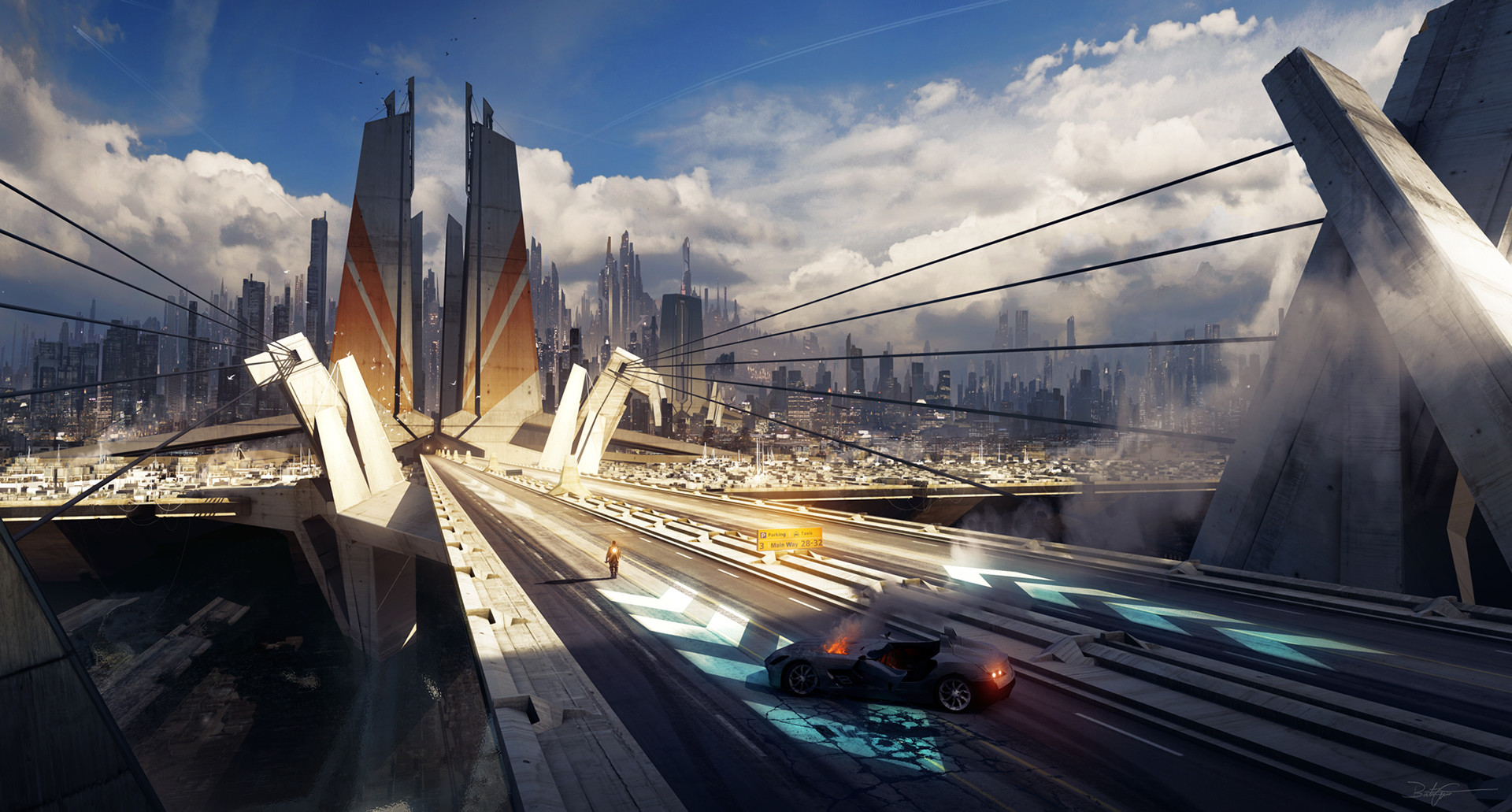The image is a still from a video game depicting a futuristic cityscape. In the foreground, there's a massive bridge supported by sturdy concrete beams and cables, extending toward a sprawling megacity on the horizon, complete with hundreds of towering skyscrapers. The sky above is a brilliant blue, dotted with fluffy clouds, emphasizing the daylight setting. The main focus on the highway is a wrecked sports car with an open cockpit, engulfed in flames at the front, with its rear taillights illuminated. There’s a lone figure, presumably the driver, who has exited the car and is walking towards the distant city. Near the car, there's a yellow sign with partially legible text, reading something along the lines of "three main way, parking 28-32, taxi." On the same highway, arrows direct traffic in both directions. The setting also features a black train with a red light, racing along the adjacent roadway, adding a dynamic element to this otherwise static scene.